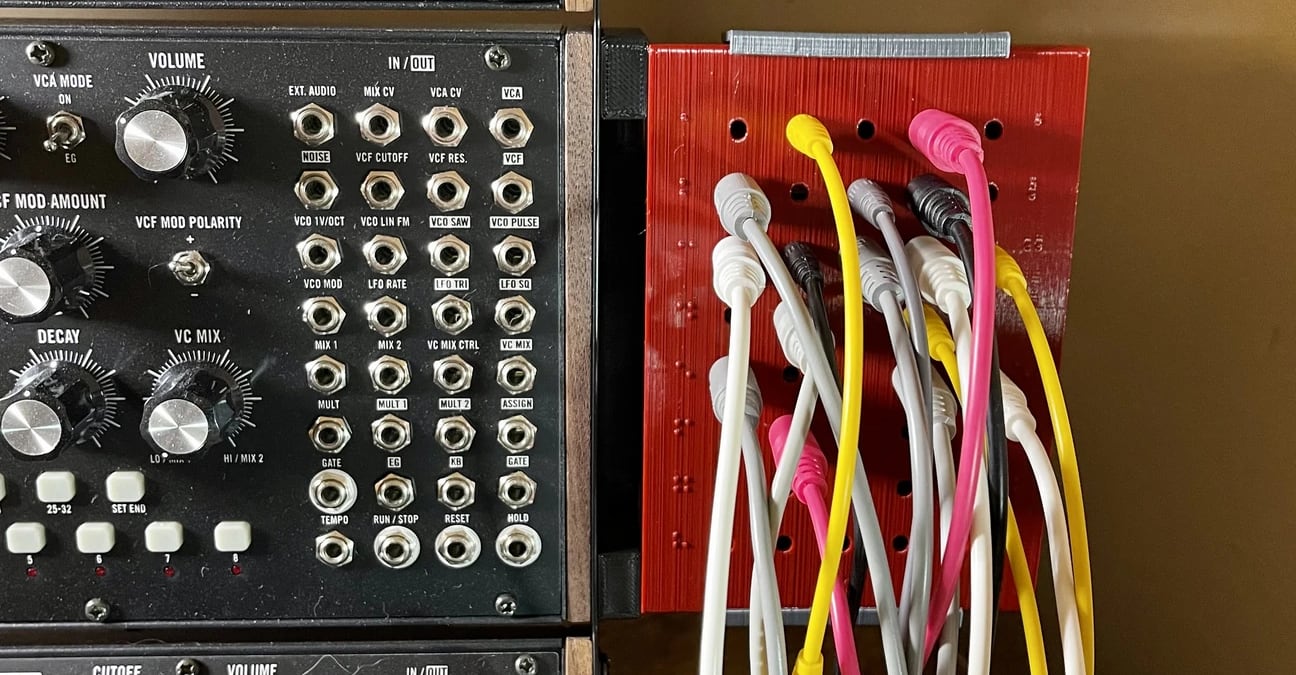This photograph captures a detailed setup of electronic audio equipment, potentially including an amplifier or a music effects board, characterized by two distinct devices side-by-side. The device on the left is a solid black rectangular unit adorned with numerous controls and labels. It features eight rows of four unoccupied ports, along with black and silver knobs labeled for functions such as "volume," "decay," "mod," and switches labeled "VCMO" and "VCF mod." White square buttons are also visible on this device. To the right, a red panel contrasts sharply, bristling with variously colored cables plugged into each of its numerous ports. This vibrant array of wires, with colors including black, red, pink, and yellow, adds to the complexity of the setup. The detailed labeling, presence of both plugged and unplugged ports, along with the vibrant, multicolored cords, suggests a sophisticated piece of audio equipment, possibly for sound modulation or mixing.